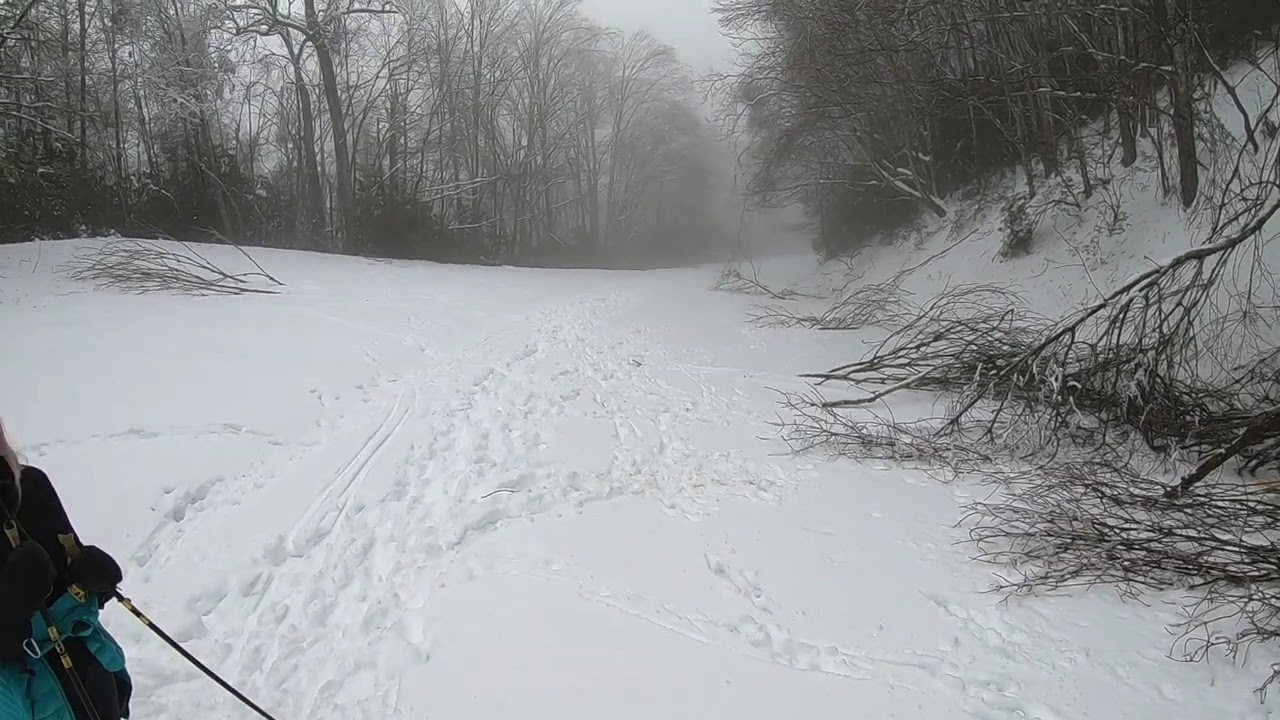A foggy, overcast scene unveils a snowy, slurry hillside, potentially within a ski resort. The foreground is marked by numerous footprints, suggesting a frequented path. Trees stand tall on both sides of the landscape, while fallen branches and thin trees litter the right side of the frame. In the bottom left corner, a person dressed in black and turquoise or greenish-blue holds ski sticks, their blue and black jacket visible above their mittens. Part of a green and black backpack with a noticeable zipper peeks into view from the lower left as well. The background dissolves into a foggy veil, enhancing the ethereal atmosphere of this serene, yet slightly desolate, wintry forest.